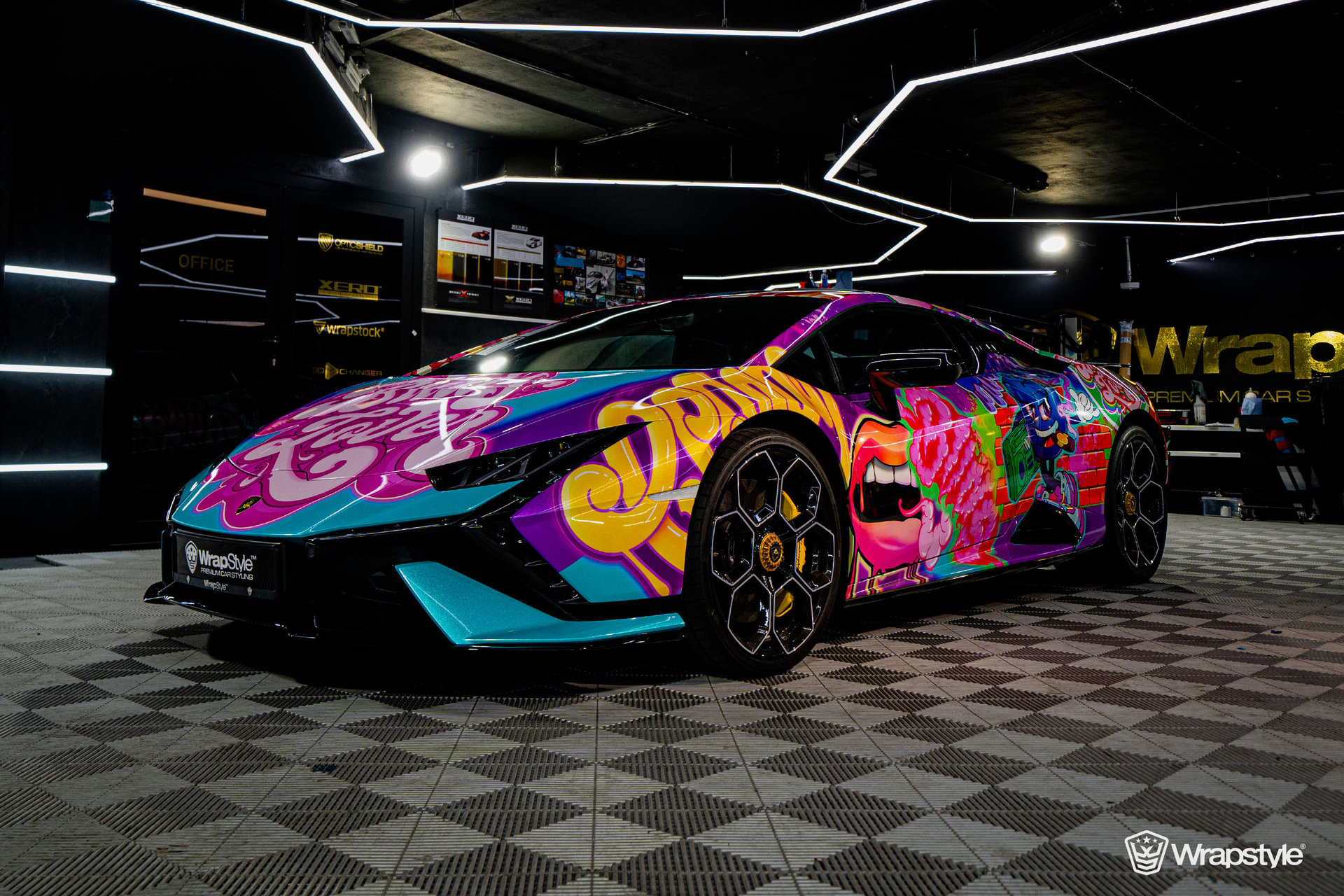The photograph captures a vibrant, futuristic sports car stationed inside a sophisticated building, possibly a high-end car garage or a dedicated wrapping studio. The car is extravagantly adorned with a wrap-style design, featuring an array of bold, cartoonish, and graffiti-like elements including an open mouth and an assortment of indistinguishable words, possibly "lover." The wrap showcases a spectrum of vivid colors, including red, pink, purple, yellow, and blue. The car's black wheels, adorned with pentagon-shaped patterns, stand out against the colorful body. The setting features a distinctive black and light gray checkerboard floor and a sleek black interior, accentuated by white geometric shapes on the ceiling and bright white lamps towards the back. Billboards and a gold logo stating “WRAP” are visible along the room's edges, reinforcing the wrap-themed atmosphere. The light gleams off the car’s low-slung body, enhancing its eye-catching appeal at the center of the image.